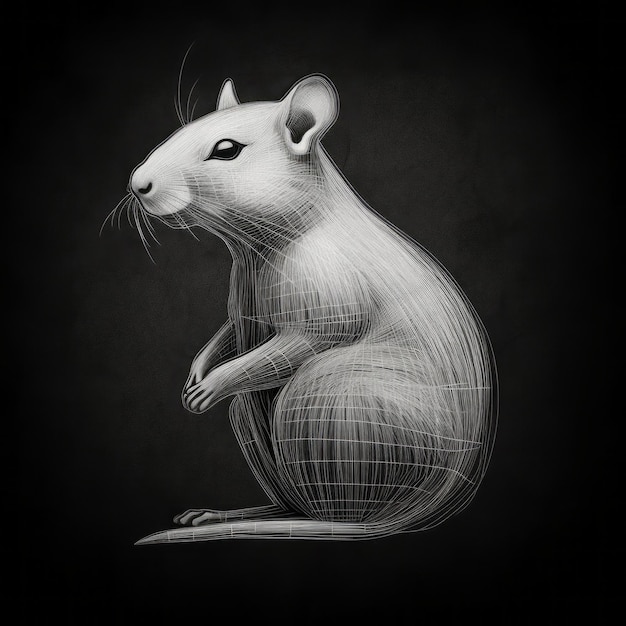This image features a meticulously rendered, computer-generated depiction of a large, gray mouse sitting upright against a completely black background. The mouse is created with intricate, hair-like strokes that give texture to its entire body. Its prominent feature includes long whiskers on both sides of its face and expressive, pointy eyebrows. The mouse's ears are small and stick out from the top of its head, while its eyes are black with a noticeable white gleam.

The creature's posture is upright on its back legs, with its forearms extended forward and paws held together. The tail, thicker and somewhat long, trails alongside its left leg, tucked next to its body rather than sticking out. The mouse's fur varies in shade, being bright white on its face and parts of its back but transitioning to a darker hue on the chest area. Despite being described as chubby and slightly hunched over, the mouse presents a tidily kept appearance with straight, well-groomed fur. The darkness of the black background starkly contrasts with the mouse's detailed and textured gray fur, making the artwork striking and visually captivating.